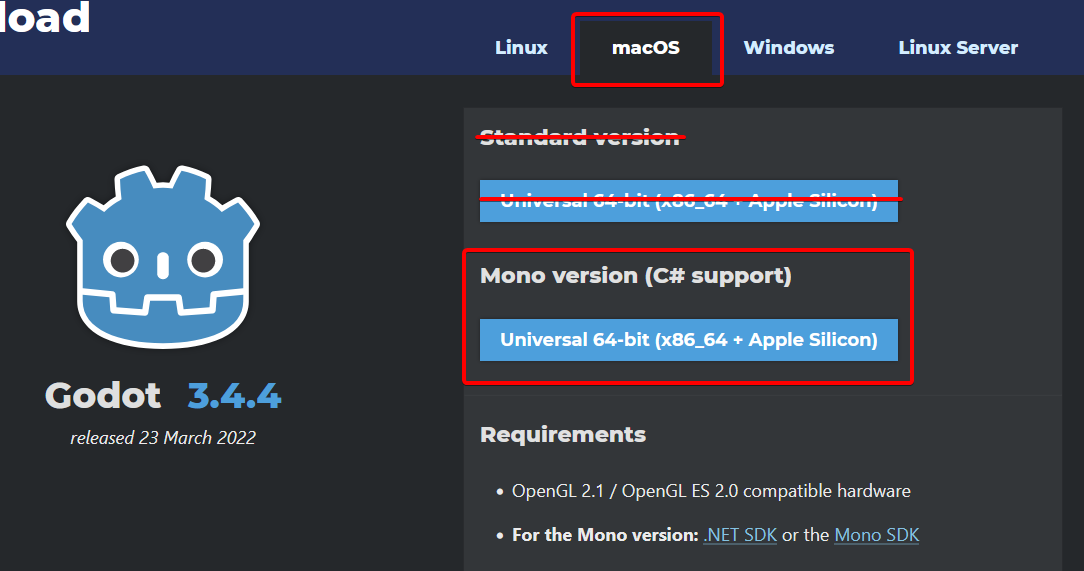This screenshot is from a website showcasing various download options for the Godot Engine version 3.4.4. The image has a dark background and features a dark purplish-blue header with multiple tabs at the top. The available tabs are "Linux," "macOS," "Windows," and "Linux Server," with the "macOS" tab selected and highlighted by a red box that appears to be added post-screenshot.

Beneath the header, "Standard Version" is written in white text on a dark grey background, but it is struck through with a red line. Below this, there is a blue button labeled "Download Universal 64-bit x86 Apple Silicon version," which is also struck through with a red line, indicating it may no longer be available or recommended.

Further down, the text "Mono Version with C++ support or C# support" is displayed, accompanied by a blue button that is highlighted with a red box, indicating this is the suggested download option. The program, Godot Engine, is identified with a blue robot head icon and the text "Godot 3.4.4," noting its release date of March 23rd, 2022.